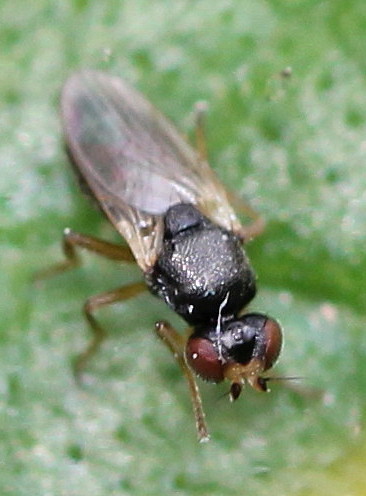This photograph presents an extremely detailed close-up view of a black fly perched on a green leaf. The fly's head, located at the bottom right of the image, features large, prominent brown eyes and two antennae or similar protrusions, likely used for feeding. Its body, observed from a front-facing angle and extending diagonally toward the top left corner, showcases a striking pattern—a black head and thorax, with hints of brown and even a touch of yellow in various areas. The fly's translucent green legs are visible; with three on the left side and one on the right, indicating the insect's slightly angled pose. The wings, tucked neatly against its body, exhibit a shimmery, light brown translucence, with sections appearing clear. The green leaf in the blurred background serves as a vibrant backdrop, emphasizing the intricate details and natural coloration of the fly.